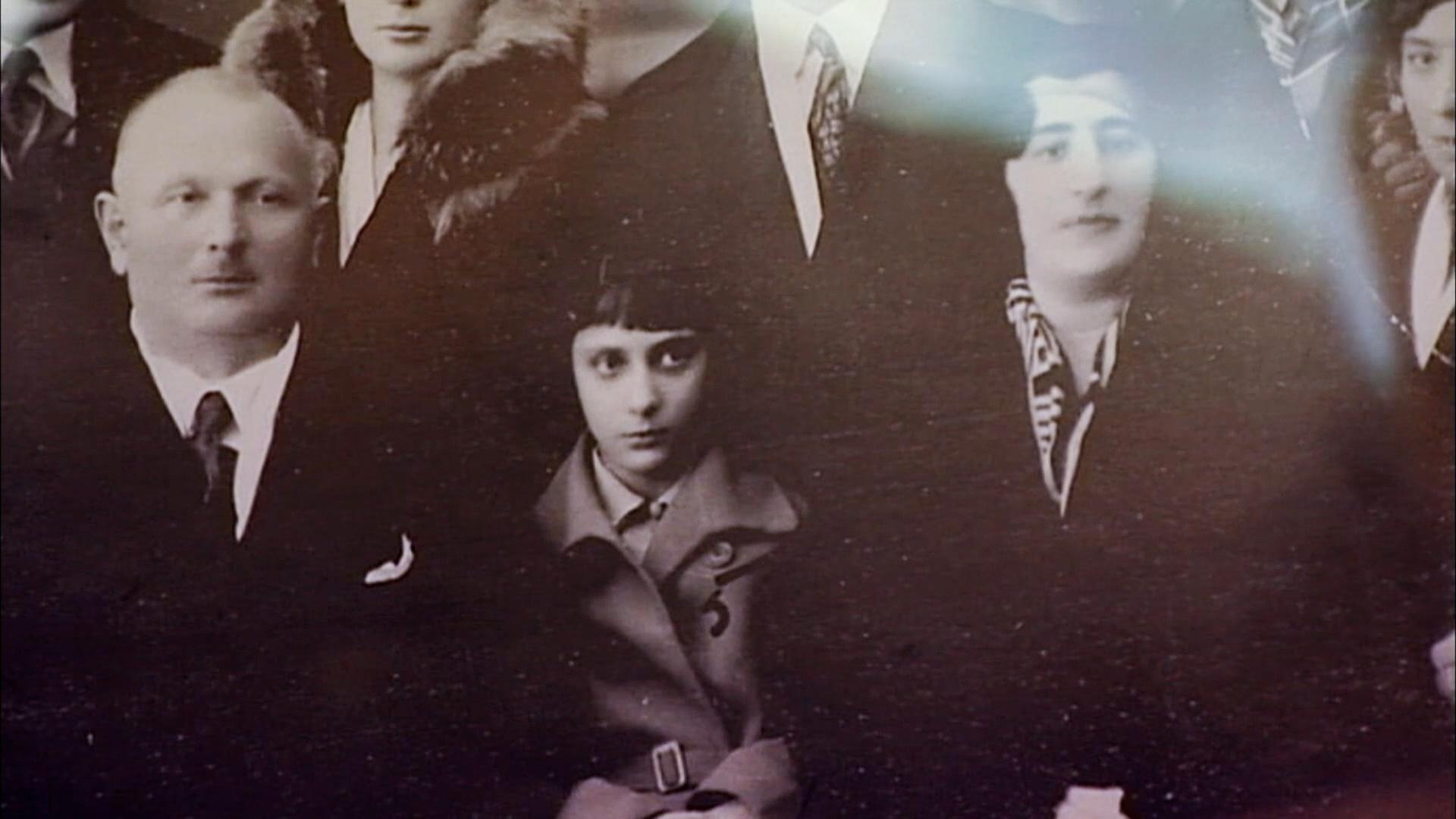This detailed black-and-white photograph captures a poignant moment from a bygone era. Positioned on the left is an older, balding man dressed in a suit complemented by a tie and a white blouse. His gaze is directed thoughtfully to the right. Adjacent to him is a younger person, possibly female, with dark hair blending seamlessly into the surrounding shadows, adding a mysterious quality to the image. This individual, centered in the composition, has wide-open eyes also looking towards the right, and is clad in a coat distinguished by large buttons, a belt, and a prominent collar. To the far right stands an elderly woman in dark attire, with only the textured pattern of her inner clothing discernible beneath the enveloping blackness. Her shoulder-length hair adds to her aged appearance. The photograph includes glimpses of other figures, whose faces and upper bodies are partially cropped out, heightening the enigmatic atmosphere. A noticeable glare occupies the top right corner, suggestive of the photo being a rephotographed print. This theory is supported by the presence of specks and artifacts, which may be dust or remnants from the original image, further accentuating its historical essence.